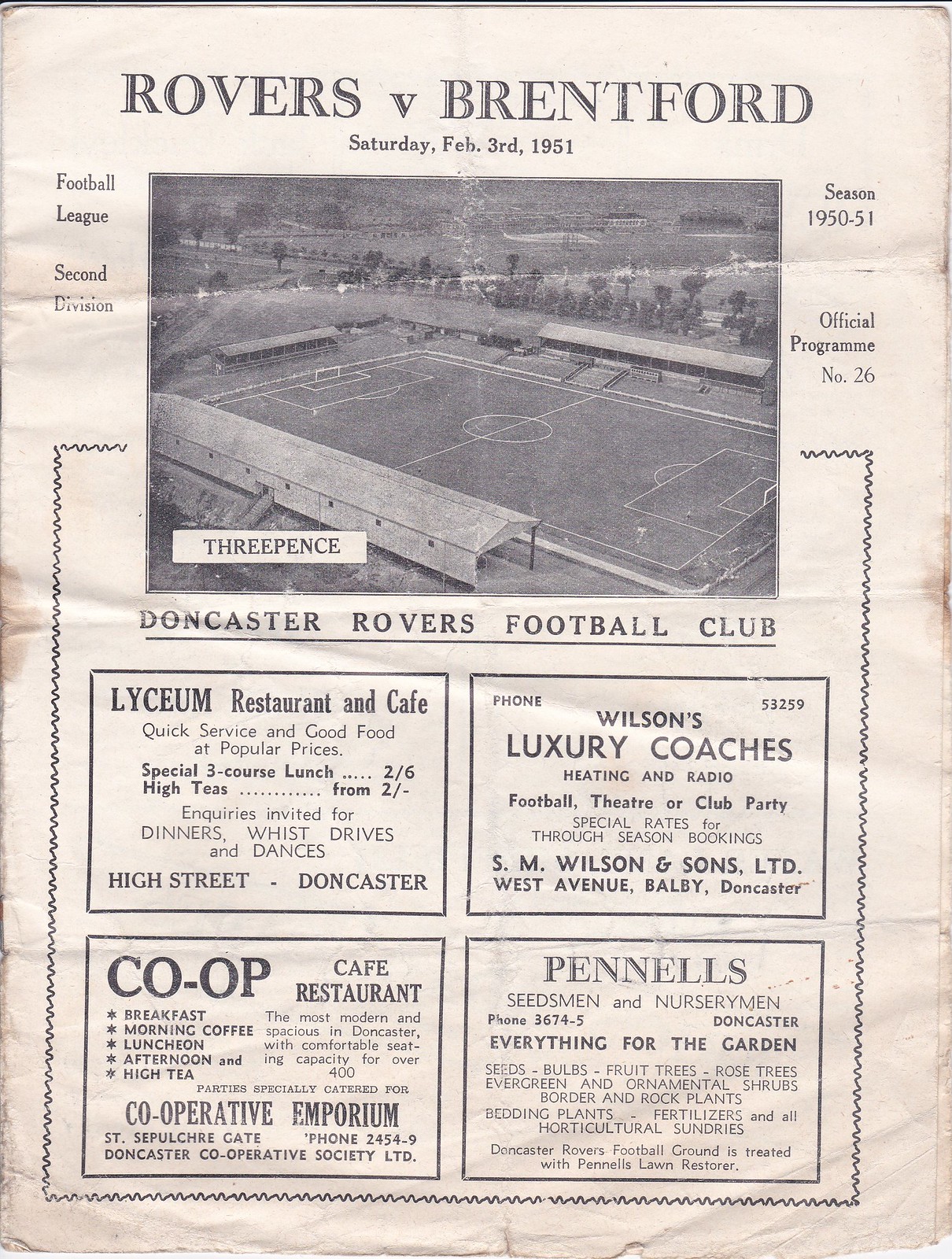The scanned image is of an old, worn-out sports program from an official Football League Second Division match between Doncaster Rovers and Brentford, held on Saturday, February 3rd, 1951, during the 1950-51 season, designated as Program No. 26. At the top, it prominently reads "Rovers vs Brentford," and "Official Programme Number 26," and below it is a 3 pence price tag. A black-and-white photograph of a deserted soccer field occupies the middle section, with the surrounding landscape in view. Beneath this image, the text "Doncaster Rovers Football Club" is displayed. The bottom half of the page contains four distinct advertisements in separate squares. The first ad promotes the Lyceum Restaurant and Cafe, offering quick service, good food at popular prices, a special three-course lunch, and high teas. The second square advertises Wilson's Luxury Coaches, emphasizing features such as heat and radio, with special rates for seasonal bookings. The third ad is for the Co-op Cafe Restaurant, noting its comfortable seating capacity for over 400 people and highlighting its breakfast, luncheon, and high tea services. The final advertisement is for Pennell's Seedsmen and Nurserymen, detailing a wide range of gardening supplies, including seeds, bulbs, fruit trees, and fertilizers, and proudly mentioning that Doncaster Rovers Football Ground is treated with Pennell's Lawn Restorer. The page captures a nostalgic snapshot of mid-20th-century football culture, complemented by the commercial offerings of the time.